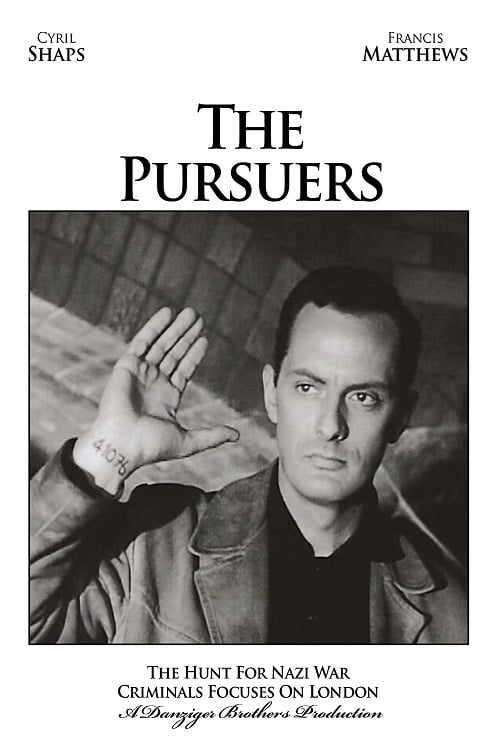The image is a black and white movie poster for "The Pursuers." At the very top of the white background, "Cyril Shaps" is written on the left and "Francis Matthews" on the right. Centered below these names, in bold black text, is the film's title: "The Pursuers." Beneath this title, occupying the central portion of the poster, is a black and white photograph of a Caucasian man cropped from the chest upwards. He is wearing a black collared shirt and a possible leather jacket. The man has short black hair, dark eyes, and dark eyebrows. He is clean-shaven and looking off to the left with a serious expression. His right arm is raised, showing a tattoo of the number "41076" on the inner wrist. Below the photograph, still on a white background, the text reads: "The Hunt for Nazi War Criminals focusses on London." At the bottom center of the poster, in cursive black text, it says, "A Danziger Brothers production."